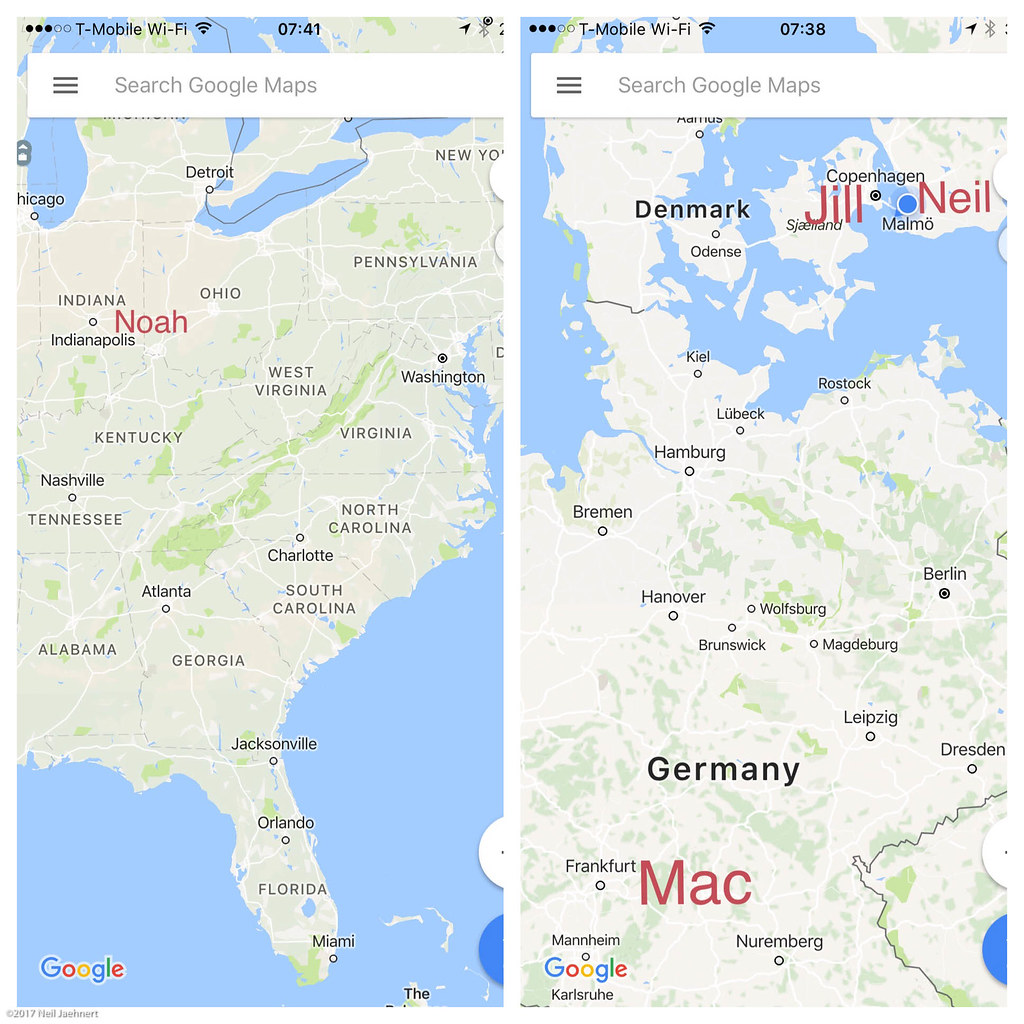The image comprises a composite of Google Map screenshots segmented into four parts, though only the bottom two sections are largely visible. The first visible map focuses on the eastern seaboard of the United States, stretching from New York down to Florida. In this depiction, parts of the Great Lakes and the Atlantic Ocean are also visible. The map uses a beige color scheme for land with green indicating mountainous regions and blue signifying bodies of water.

The second visible map covers a portion of Europe and prominently features the text "MAC" in large red letters, along with the Google logo beneath it. This map includes parts of Germany and Denmark, with specific cities such as Copenhagen clearly labeled. Additionally, in the upper right-hand corner, "Jill Neal" is highlighted in big red letters. Various regions within Germany are also distinctly marked alongside two specific locations within Copenhagen, providing a comprehensive geographical context.